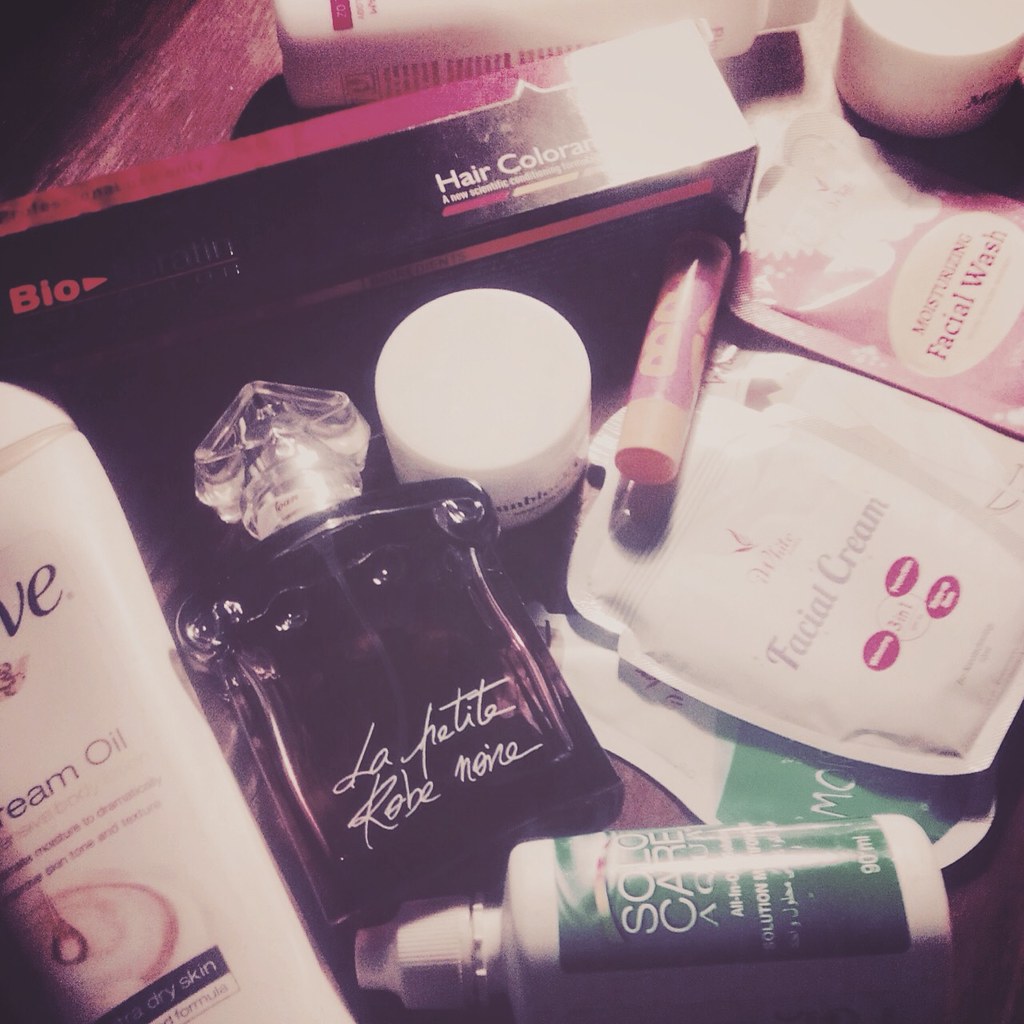The close-up image showcases an assortment of beauty and skincare products arranged on a worn dark wooden tabletop. On the left side, there's a white bottle of Dove Cream Oil, specifically formulated for dry skin. Adjacent to it is a perfume bottle with a clear glass top and a purplish-pink hue. The label reads "La Petite Robe Monet." Above the perfume sits a black hair color box with red detailing.

Directly beneath the hair color box, there's a partially obscured white circular container, the label of which is not visible. To the right, a collection of colored chapsticks rests on top of a pack of facial cream that is predominantly white. This pack, in turn, is placed over another pack that is white and green, though the contents are indistinguishable.

In the bottom section of the image, there's a white and green bottle that appears to be eye contact solution. In the upper right corner, a pink packet labeled "Moisturizing Facial Wash" is visible. Above this packet, yet another white circular container is positioned, adding to the diverse array of beauty items captured in the image.